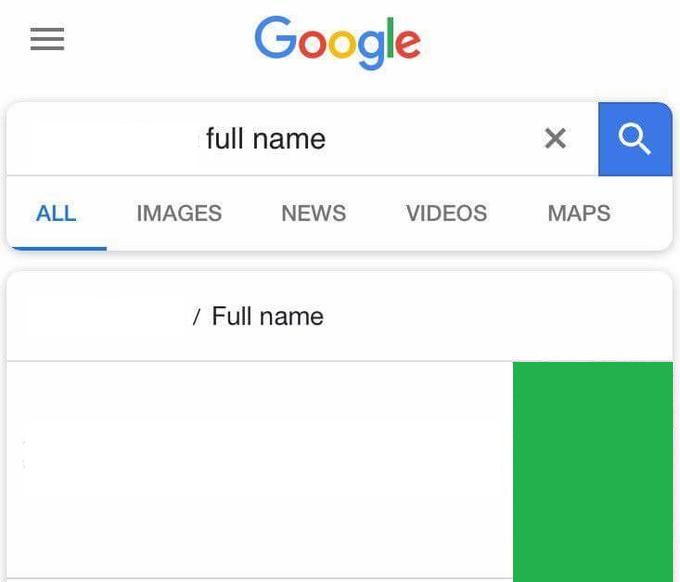The image displays a Google search page. On the top left corner, there are three horizontal lines in gray. To the right, the Google logo features a capital blue "G", followed by a red "O", yellow "O", lowercase blue "g", green "l", and a red "e". Below the logo, there's a search bar with a white background. Inside the search bar, the text "full name" appears in black, small lowercase letters. 

Next to the right of the search bar, there is a gray "X", followed by a small blue square containing a white magnifying glass icon. Beneath the search bar, a horizontal gray line spans across. Below this line, a white box displays the word "ALL" in blue, capital letters, and a blue underline highlights it. 

To the right, other search categories are listed: "IMAGES" in gray capital letters, followed by "NEWS", "VIDEOS", and "MAPS", all in similar gray capital lettering. Further down the page, there is another white box containing the text "\ full name", with "F" capitalized and "ull name" in lowercase black letters. Underneath this, there's another blank white box, and to its right, a green box with no content inside.